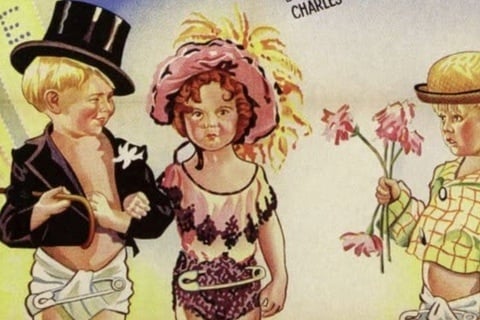The image depicts an old-style, hand-drawn cartoon, reminiscent of illustrations from the 1950s, possibly from a magazine or pamphlet. It has a slightly eerie vintage charm. The scene includes three babies dressed in whimsical adult attire, arranged against a yellowish-white background with some indistinct brightening.

On the left, a Caucasian baby boy with blonde hair is dressed in an ensemble mimicking a tuxedo, including a shiny black top hat tilted to one side and a tuxedo coat cut above his diaper. His diaper is pinned at the front, and he's holding a cane or umbrella in his right hand, smiling at the baby girl next to him. The girl, with red hair and pale skin, wears a large pink hat adorned with yellow feathers and a pink dress featuring purple flowers. She has her arm entwined with the boy's, accentuating the playful adult mimicry.

To the right of the girl, another baby boy stands, wearing a yellow shirt with an orange checkered pattern and an orange wicker hat. He holds flowers with green stalks and pink petals in his right hand. Like the others, he has his diaper pinned at the front and his belly showing. The overall composition humorously portrays the toddlers as if engaged in adult roles, creating a scene that is both whimsical and quaintly nostalgic.